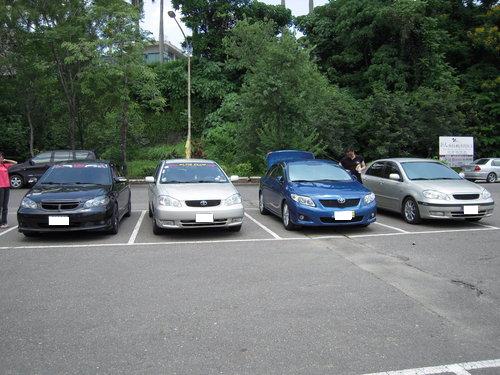In this landscape-oriented photograph, we see a parking lot with four sedans parked perfectly within the lines, all facing the same direction. The vehicles from left to right include a black compact SUV with some sort of words on the windshield, a silver-gold colored sedan, a darker blue sedan with its trunk open, and another sedan in a creamy or champagne color. In the background, lush green trees form a dense forest backdrop. On the far left side of the image, another SUV is partially visible. A woman in a pink shirt and black pants stands slightly out of focus on the left-hand side, her left arm hanging through the picture. Between the third and fourth cars, a man in a black t-shirt is seen looking into the driver's side window of the creamy sedan, holding something in his left hand. In the top right corner of the photo, another vehicle can be seen driving off near a sign for a local business.